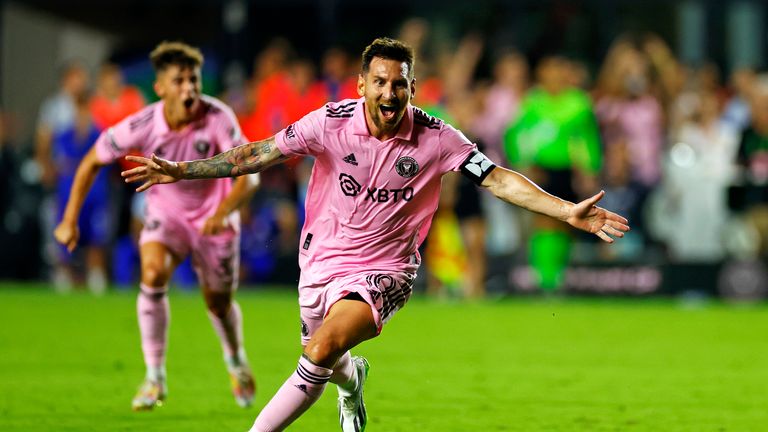The image captures an ecstatic Lionel Messi celebrating a goal on a green soccer field. He is at the center of the photograph, clad in a pink jersey with black stripes, a collar, and various logos, including “XBTO” visible across his chest. He pairs this with white shorts featuring black stripes, knee-high white socks, and white cleats. Messi's distinctive sleeve tattoo adorns his right arm, while his left arm is visibly clear. His short brown hair and beard stubble are noticeable, and he has both arms extended outward, exclaiming in jubilation. Behind him, a teammate wearing the same pink attire is also celebrating, his expression animated as he runs in the same direction as Messi. The background features a blurred crowd dressed in bright colors, emphasizing the focus on Messi and his teammate in the foreground.